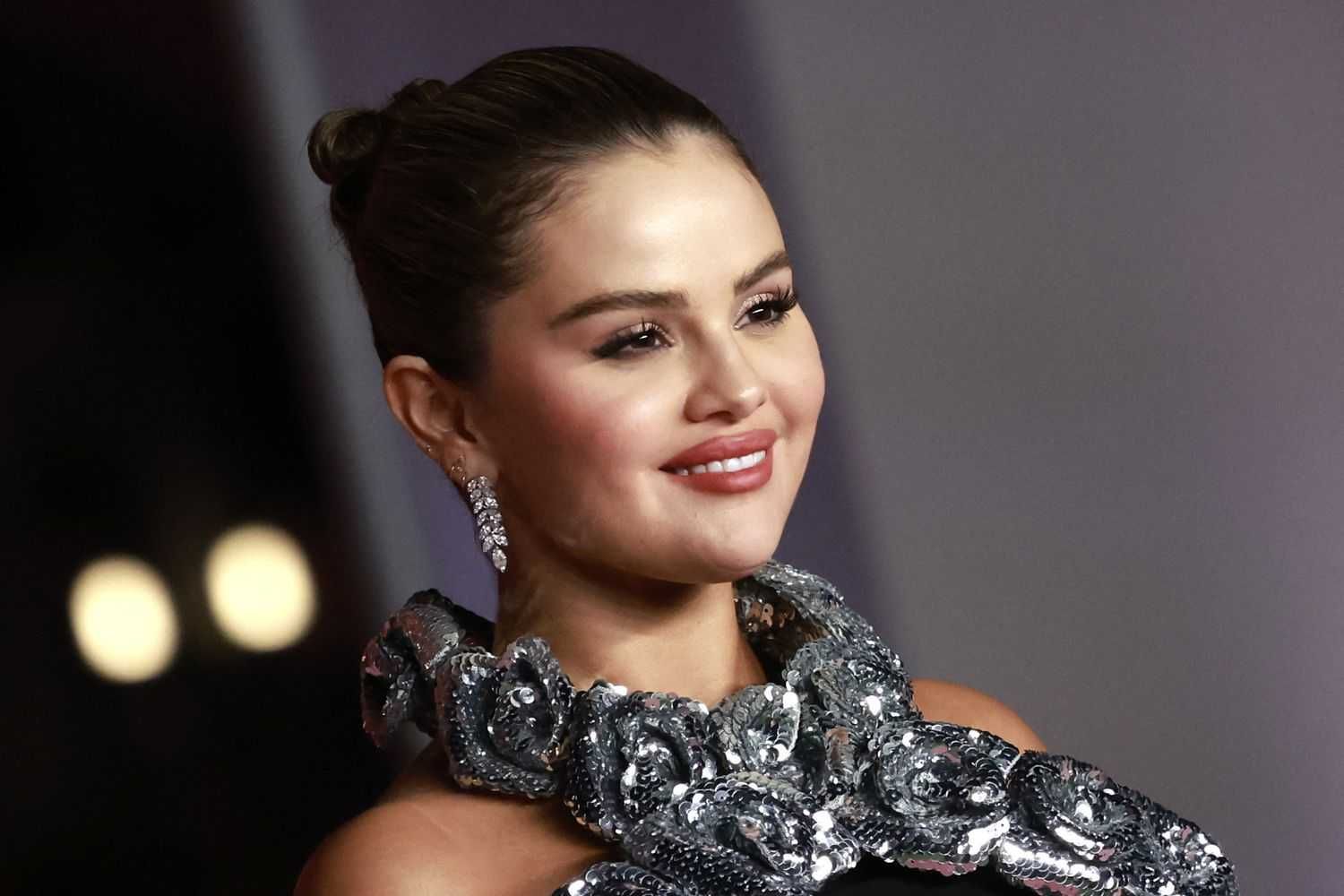This photograph captures a young woman, seemingly Selena Gomez, dressed in an elaborate and celebratory outfit. Her hair is styled in a sleek bun, revealing her lustrous black hair. She is adorned with long, dangling diamond earrings that gleam with sophistication. Her dress, or more precisely the neck area of her attire, is particularly noteworthy; it features an opulent, silvery, shimmery design that is thick and ornate, almost resembling a wreath. The dress itself appears to be black, though only the shoulders and a portion of it are visible in the shot. Selena's complexion is tan, and she wears a broad, self-assured smile. The background is a simple grey wall, illuminated by two stage lights positioned to the left of her, suggesting she is at a high-profile event or Hollywood gala. Her poised demeanor and intricate attire underscore her celebrity status.